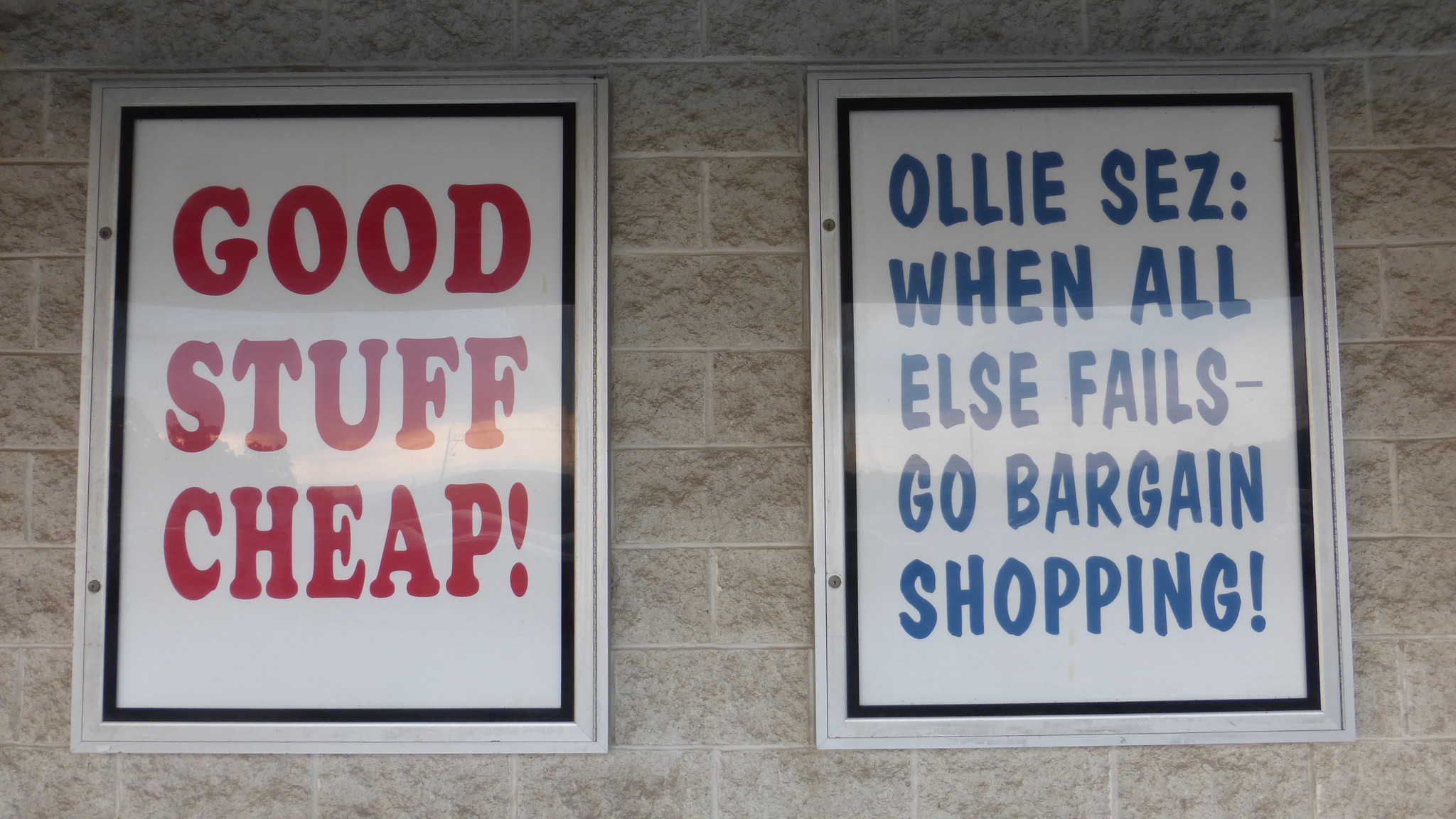The image captures an indoor stone wall constructed of beige-gray stone bricks arranged in a standard brick pattern, with visible mortar between the stones. Illuminated solely by natural light, the scene feels serene and subtly lit. Affixed to this rustic wall are two rectangular signs, each taller than they are wide, with an approximate height-to-width ratio of 60:40. Both signs are enclosed in sleek silver frames with black interior linings. 

The left sign features a white background with bold, red capital letters that read: "GOOD STUFF CHEAP!" The right sign, also set against a white background, displays the text: "SCZ: When all else fails - go bargain shopping!" Each sign stands out prominently against the stone wall, conveying a sense of thrifty enthusiasm and pragmatic advice.